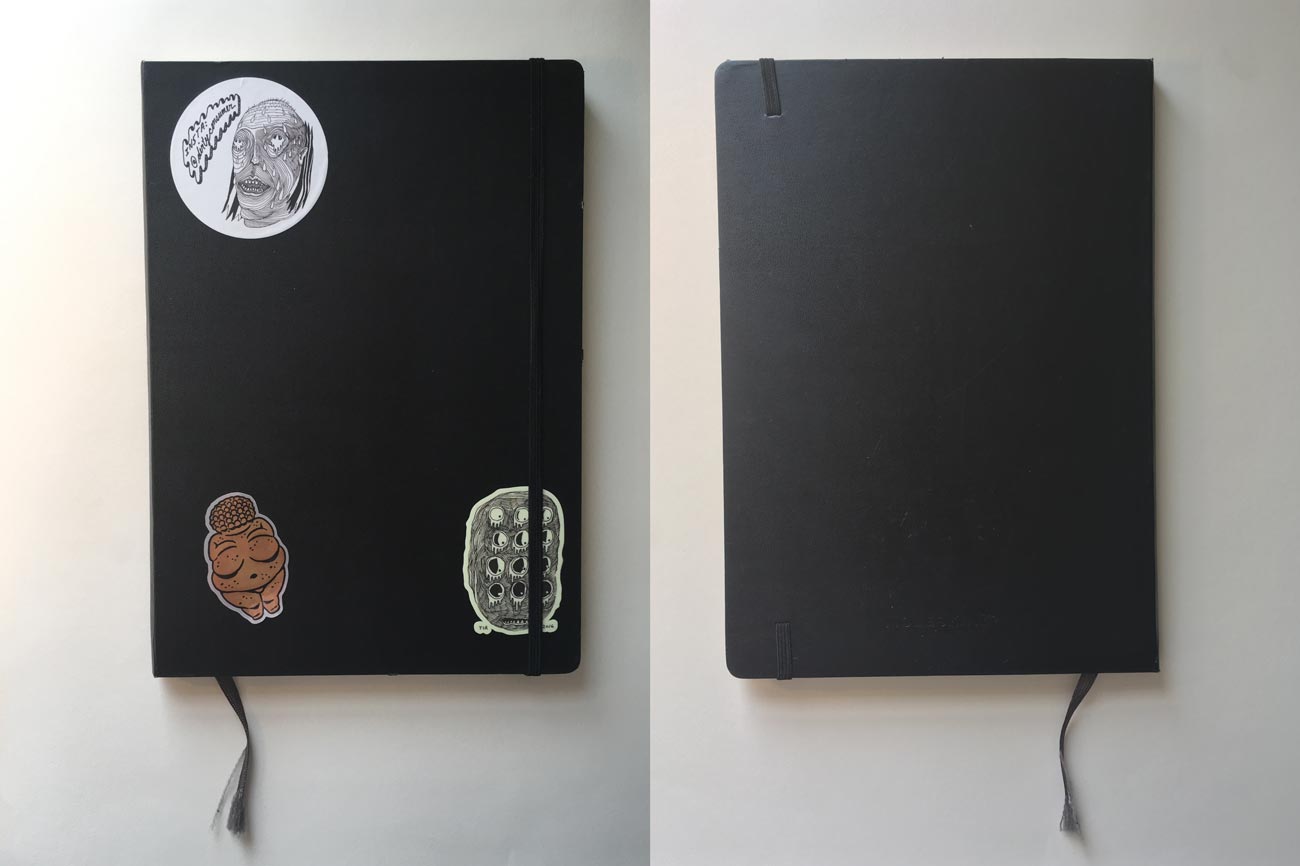The image showcases two photographs of the same black square notebook against contrasting backgrounds of light gray and dark gray. The left photograph presents both the front and back covers of the notebook side-by-side, while the right photograph focuses on the front cover. The notebook’s front cover features three distinct stickers: The top left sticker is round and grayscale, depicting a stone-like face with hollow eyes and hair trailing from the temples to the back of its ears. The bottom left sticker shows a Buddha figure in a terracotta color. The bottom right sticker is also round, featuring a whimsical, furry creature with four sets of eyes arranged in three rows and an expressive mouth. The back cover of the notebook is entirely plain black, with no stickers, save for a small black string bookmark at the bottom. The overall composition effectively highlights both the decorative front and the minimalist back of the notebook.